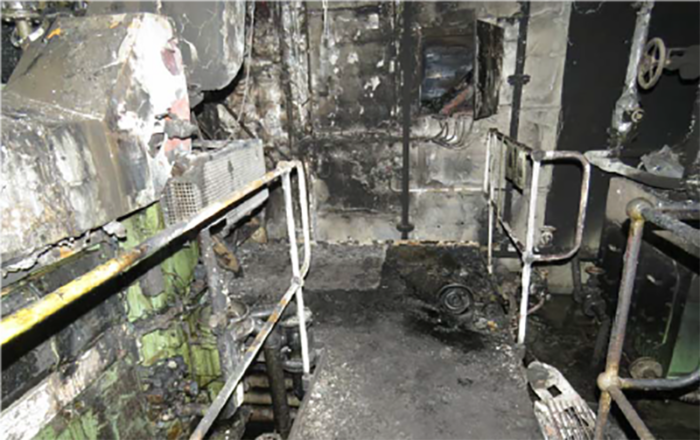This photograph captures the aftermath of a devastating event in what appears to be an old, burned manufacturing facility. The interior, covered in a thick layer of black soot, reveals equipment and machinery in varying states of decay and destruction. On the left side of the image, there is a partially visible piece of machinery, originally light green but now grimy and blackened, with pipes extending from it. The middle of the photo shows a narrow, elevated walkway bordered by railings, suggesting this could be a catwalk or slim platform, possibly above a drop. To the right, large wheels that look like valve turners are visible along with a vertically positioned pipe and a steering-wheel-like valve. Concrete walls, appearing heavily damaged and darkened, frame the scene, enhancing the bleak and monochromatic ambiance. Rust, grime, and burnt remnants are prevalent throughout, giving an impression akin to a setting from a horror movie.